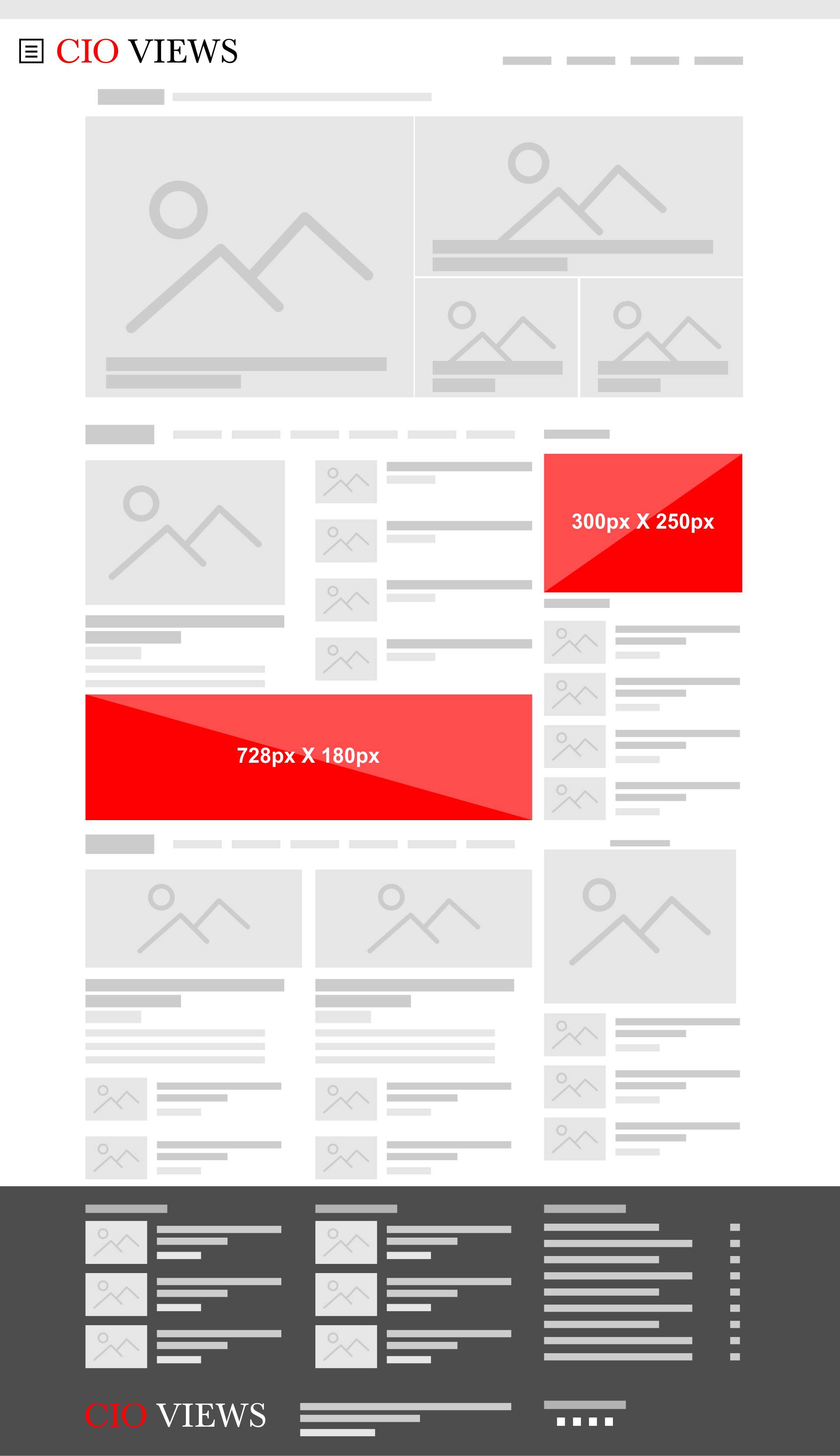The image appears to be a screenshot with a vertical orientation and a predominantly white background. It is divided into two main sections. The top section features elements in gray and red, while the bottom section is a darker gray, nearing black.

In the upper left corner, the red text "CIO" is prominent, followed by "views" in black. Below this, a gray rectangle contains a series of simple graphics: mountain-like triangles with a circle to the left, symbolizing the sun. There is a large version of this graphic on the left, and on the right, a smaller version at the top, followed by even smaller versions in two squares at the bottom.

Moving to the next section, there is a small square repeating the same mountain-sun graphic. Columns around this graphic seem intended for text, suggesting a layout or template.

On the right side of the image, a red box displays the dimensions "300px by 250px." Towards the bottom center, another red, rectangular box reads "728px by 180px." Finally, at the bottom, there are three columns with squares and bar-like graphics, indicating lines of text. The phrase "CIO views" appears again at the lower section of the image.